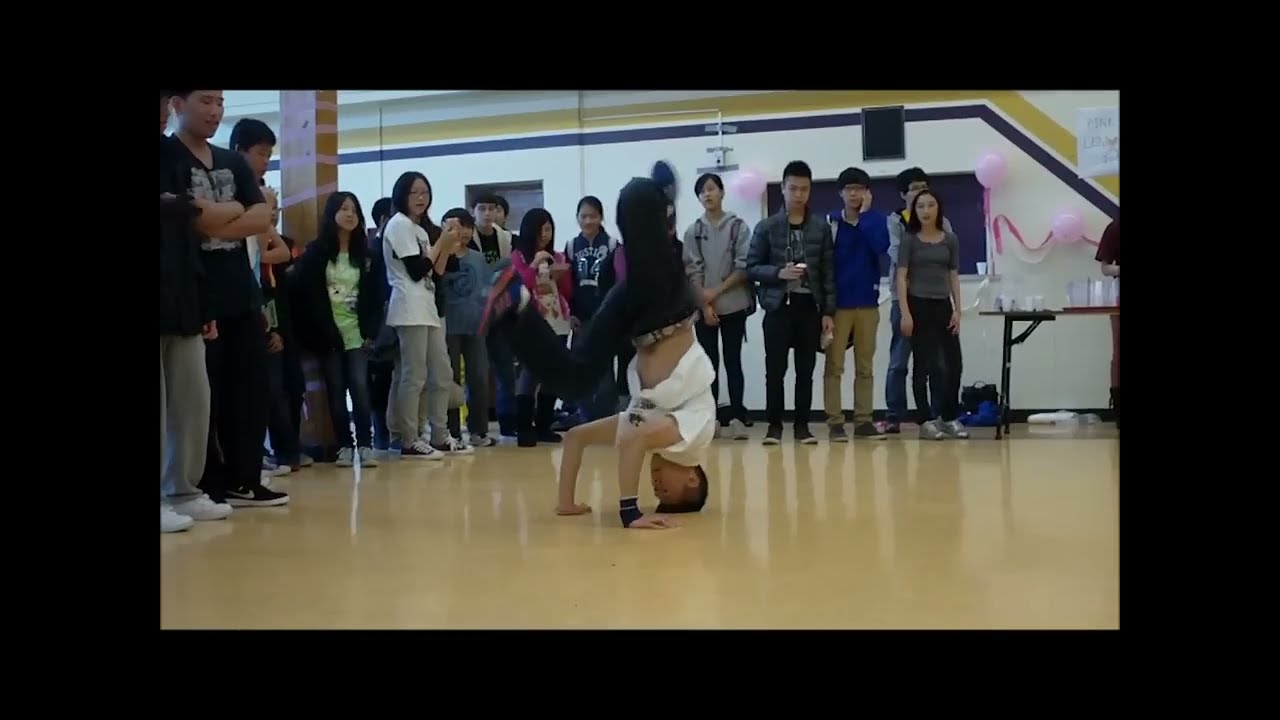In a bright, reflective gymnasium with a glossy light brown floor and a white cinder block wall accented with blue and gold stripes, a young man performs a headstand at the center of a semicircle of spectators. The observers, likely high school or college students of Asian descent, are dressed mostly in jeans and t-shirts, their dark hair framing faces filled with curiosity and excitement. The headstanding performer, clad in a white shirt that's lifted due to his inverted position and black pants, appears to be mid-motion, suggesting a possible breakdancing maneuver. One of his legs is bent downward while the other is bent at the knee, adding to the dynamic feel of the scene. To the right side of the image, a table with various glasses, possibly containing water, is visible. The photograph, bordered in black, hints at being a still from a video, capturing the energetic atmosphere and the keen focus of the young audience.